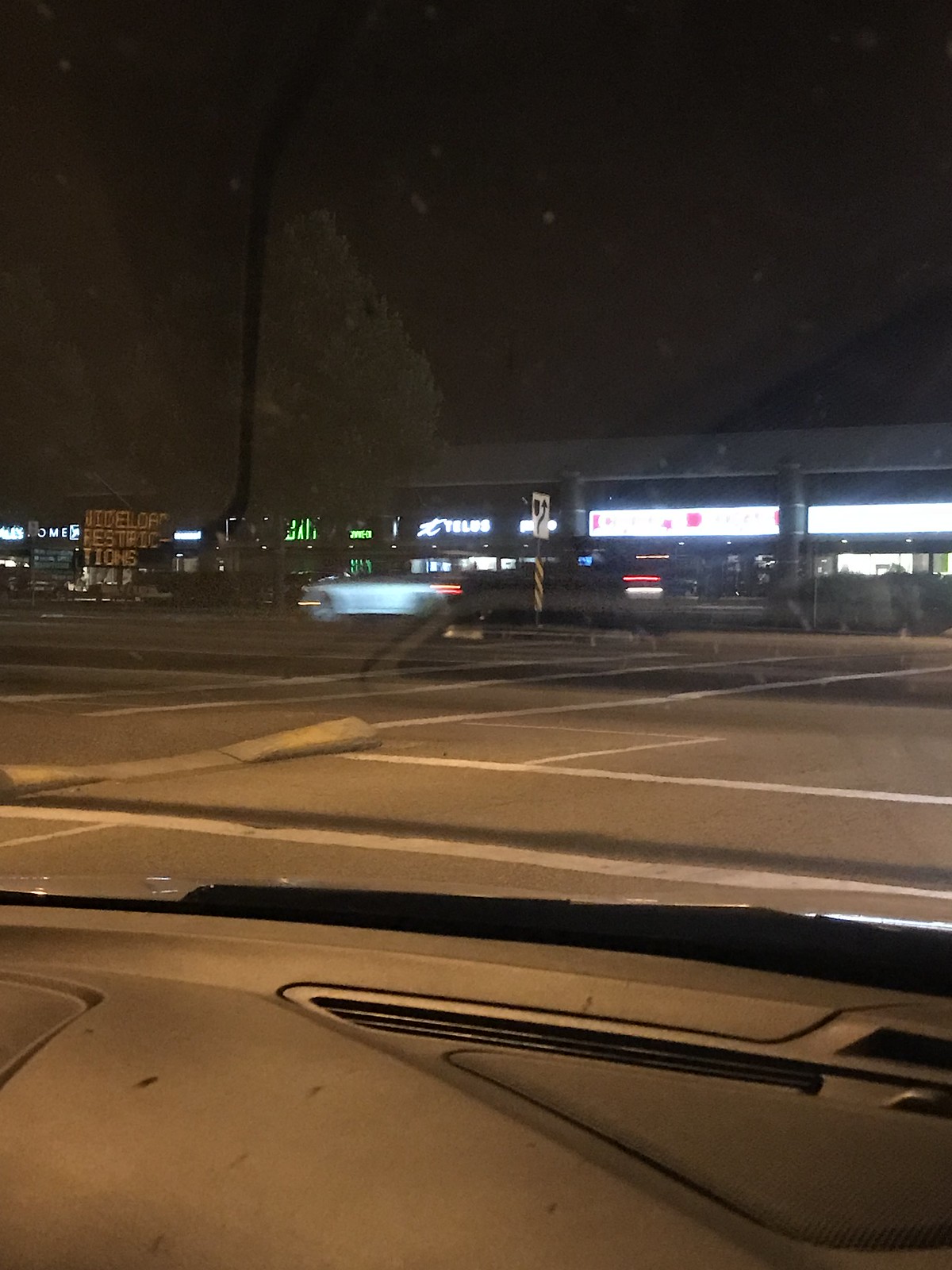The image, captured at night from inside a vehicle, showcases an outdoor scene through the windshield. The lower quarter of the photo reveals the car's gray interior, featuring a speaker on the left and air vents at the bottom. Outside, a dimly lit parking lot with visible white lines extends into the background. The dimly lit scene suggests it’s evening time, further darkening much of the environment. 

In the distance, a roadside electronic sign with yellow text, partially readable as "something ride something restrictions," can be spotted. Adjacent to it is a shopping center decorated with numerous neon signs, one of which reads "TELUS". The storefronts, although recognizable, remain blurred and indistinct. On the left side of the image, a tree’s leaves add a touch of green to the otherwise dark scene.

The road ahead is visible, with cars moving, their headlights and brake lights streaking through the darkness. A white truck can be identified towards the center-left of the image. The entire backdrop is marked by a blend of artificial lights and the obscurity of the night sky, encapsulating a mundane urban moment.